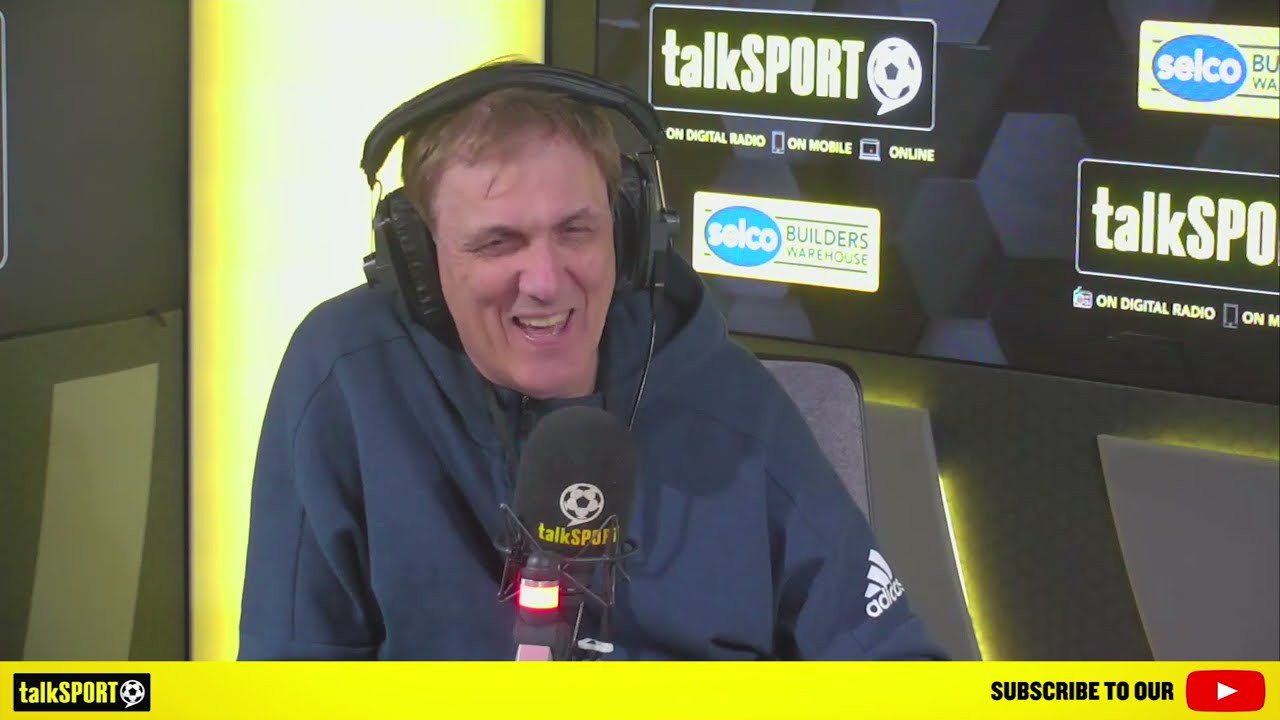This is a detailed screenshot of a YouTube video showing a still image of a podcast. Centrally featured is a man with light skin, who has sparse brown hair and prominent facial features, including a noticeable nose and cheekbones. He is wearing a blue Adidas jacket or hoodie, identifiable by the Adidas logo on his left arm, and over his ears, he has bulky, padded headphones. His mouth is open, showing his top teeth, giving the impression that he is talking or possibly laughing, with his eyes slightly crinkled in a smile. 

In front of him, there is a microphone emblazoned with the word "Talksport" and a football logo. Part of his green chair is visible. Behind him, a large screen displays repeating text and logos, including "Talksport," "Selco Builders Warehouse," and promotional phrases like "on digital radio, on mobile, online," in white, green, and yellow colors.

At the very bottom of the screenshot, there's a yellow horizontal strip. On the left side of this strip is the Talksport logo, and on the right, the text reads "SUBSCRIBE TO OUR," followed by the YouTube icon, which is a red rectangle with a white play button in the shape of a triangle.